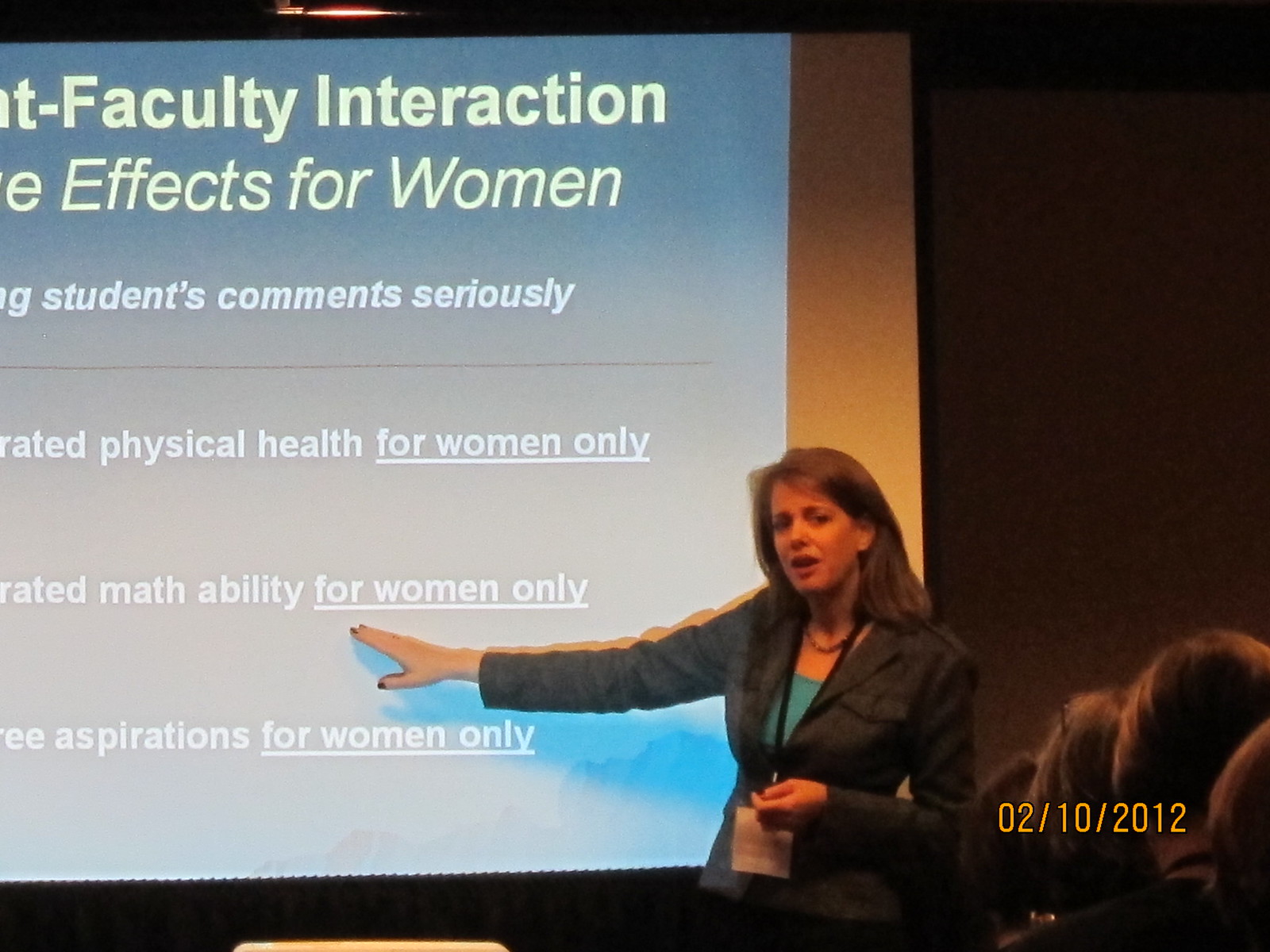In the image dated February 10, 2012, a woman with shoulder-length hair is seen giving a presentation in front of a partially visible projection screen. She is dressed in a dark suit or jacket paired with a light blue shirt and is wearing a lanyard with an identification card around her neck. Her right hand is extended towards the screen, which displays a PowerPoint slide with text in white on a gray background. The visible text reads "Faculty Interaction Effects for Women," followed by phrases such as "Students Comment Seriously," "Physical Health for Women Only," "Math Ability for Women Only," and "Aspirations for Women Only," with "for women only" being underlined in each instance. The image is taken from behind the audience, capturing the backs of four audience members' heads, indicating she is speaking to a group of people likely about issues affecting women. The woman's left hand is positioned in front of her body, and her mouth is open, suggesting she is actively speaking.